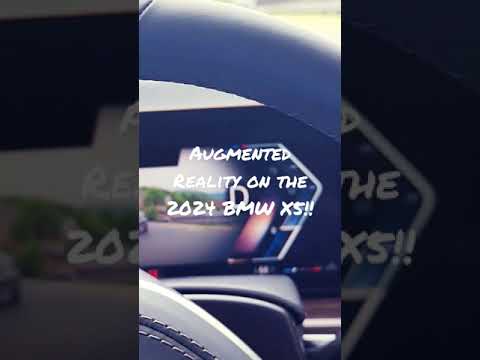This vertical image captures an extreme close-up of the steering wheel and dashboard of a 2024 BMW X5, clearly taken from the driver's perspective. The top of the image prominently displays the round upper section of the steering wheel, wrapped in black leather with distinctive white stitching. The bottom left corner reveals a small segment of the steering wheel's central hub. Behind the wheel, the dashboard is visible with a bluish-gray hue, featuring a colorful LCD screen in the gauge cluster area. The screen shows an image of the car driving down a road and includes a large, white "D" indicating the vehicle is in Drive mode. Above the screen, text has been overlaid, reading "Augmented Reality on the 2024 BMW X5!!", emphasizing the advanced technology in this vehicle. The scene is well-lit, indicating it was taken during daytime, capturing a sleek and modern interior design with a mix of black, gray, white, blue, green, and orange colors.